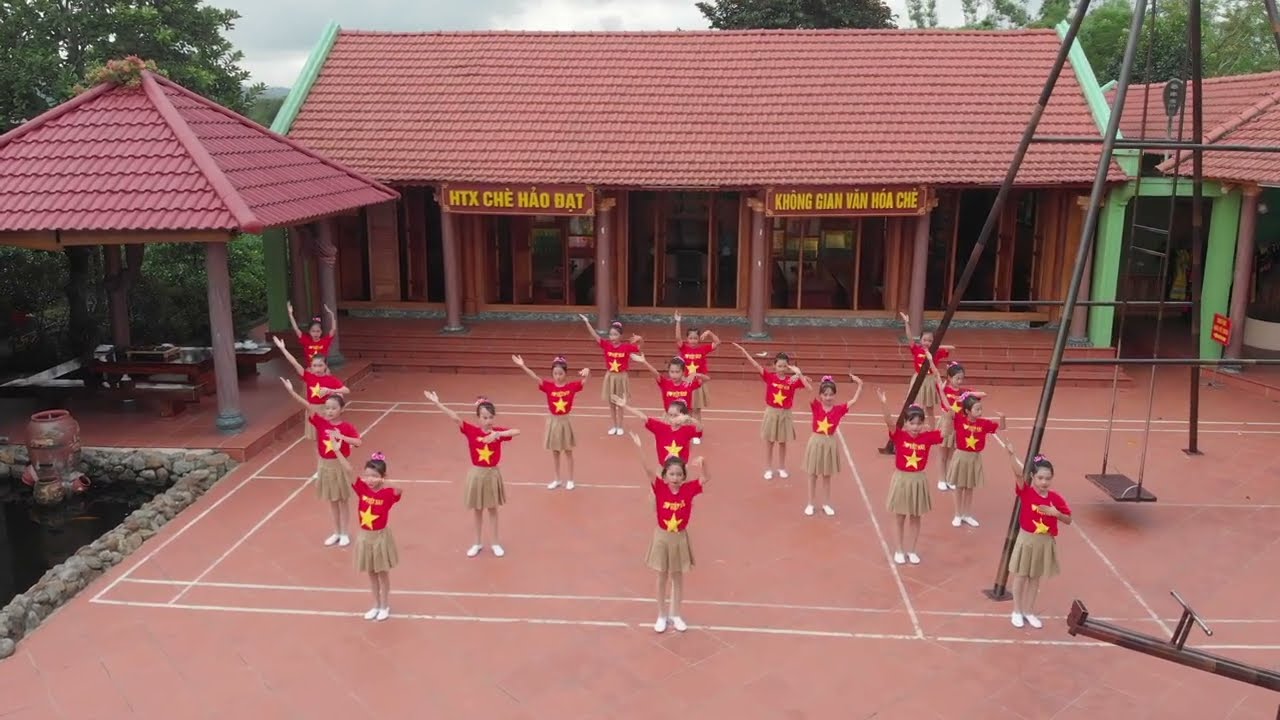The image is a photograph taken on a bright day, showcasing what appears to be a cheerleading camp or routine taking place on a clay-colored cement area, possibly a repurposed tennis court. In the foreground, there are at least 20 young girls, likely between 8 to 10 years old, dressed identically in red shirts adorned with yellow stars and some unreadable text, brown skirts, and white sneakers. The girls are arranged in a V formation with a group on the left, a group on the right, and four girls standing in a line between them, all extending their right arms out to the left as part of a synchronized dance or cheer routine. Behind them is a structure with several large windows and an orange-to-red tiled roof, featuring Chinese text above each door. To the left, there's a canopy area with a red triangular roof, possibly a picnic or rest area. The overall setting suggests a lively and organized event, possibly on a school campus.